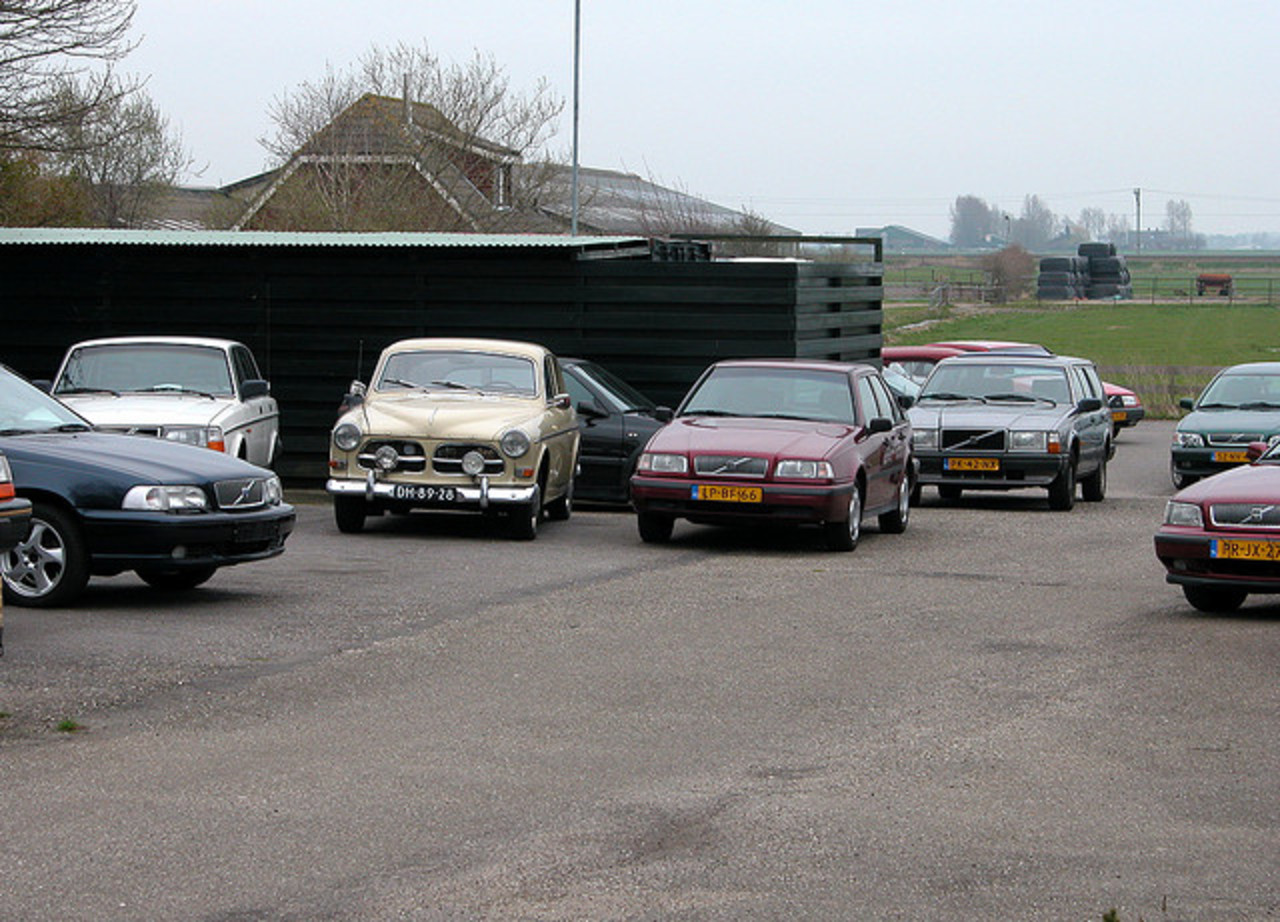The image captures an outdoor car parking lot filled with numerous vehicles, primarily older model Volvos, likely from the 90s, facing the viewer with long, yellow European-style license plates. Around ten cars are visible, including blue, white, red, green, beige, gray, and black color variations. On the left side of the image, partially hidden behind a tree, is a distinctive green car, while to its right, sequentially parked, are several others: a white car, a beige car with a black vehicle behind it, and a red car with an orange license plate featuring black letters. Midway through the parking lot, a lighter green car and two more red cars are noticeable, with another red car and green car positioned in the right foreground.

In the background is a green wooden structure with a rectangular shape and a nearly flat tin roof. Beyond this structure lies a farm, identifiable due to the green fields and scattered metal fences, some black objects or tires on the ground, and occasional hay bales. Notably, a multi-story house with red walls and a brown, pyramid-shaped roof partially obstructed by leafless trees extends to the horizon. The far background is decorated with various trees and a clear light blue sky, contributing to the overall serene yet detailed rural setting.